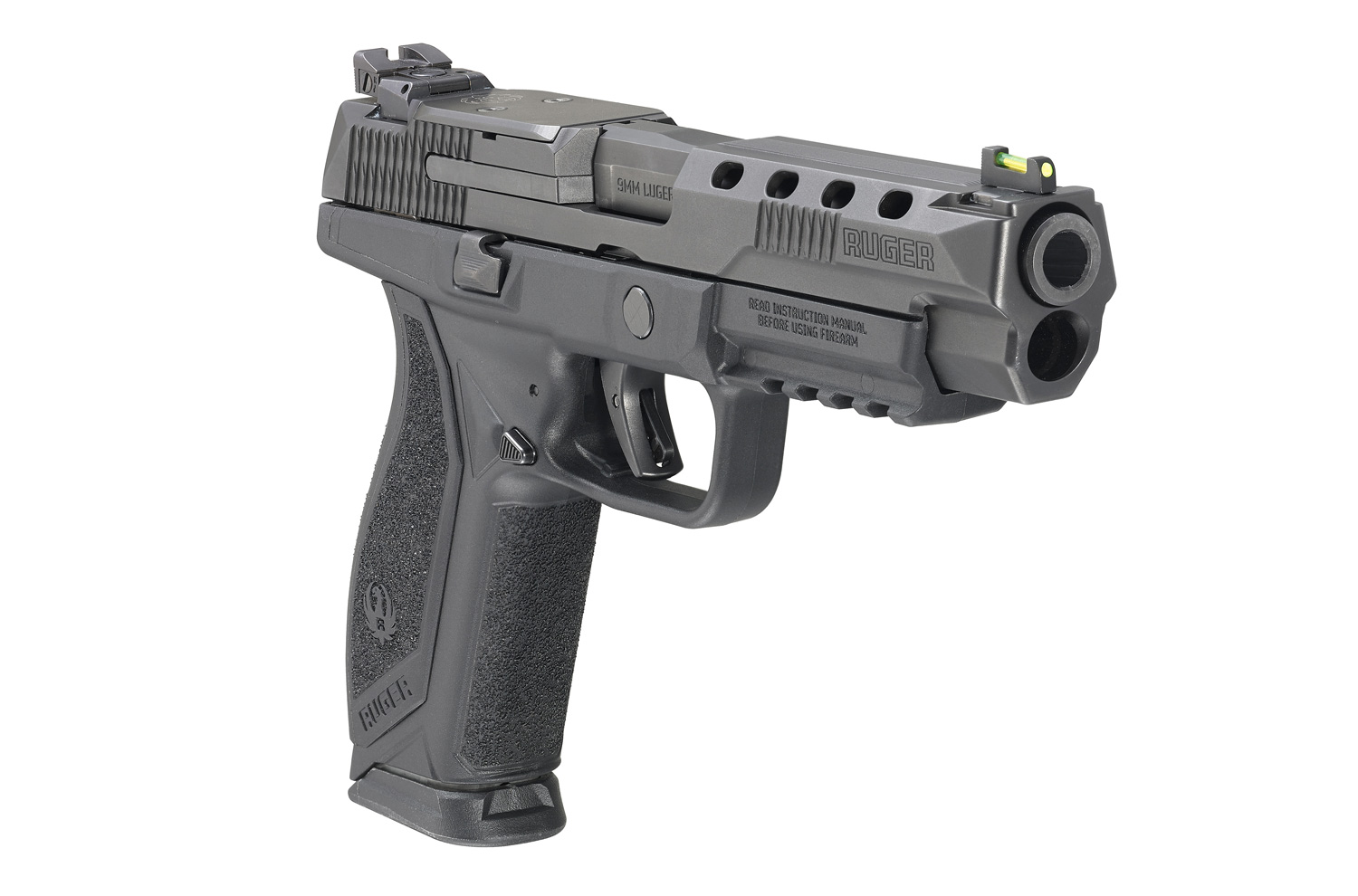The image depicts a detailed side view of a Ruger 9mm pistol, rendered in a classic steel blue color with a black, no-slip grip handle. The barrel, pointing to the right, features two internal holes and prominently displays the brand name "Ruger" in carved letters at the front. Situated just behind the muzzle, the sight incorporates yellow and green elements for improved aiming accuracy. On the underside of the barrel is an inscription advising users to read the instruction manual before operating the firearm. The handle is robust, adorned with another Ruger logo, and includes a safety trigger on its side. The magazine clip is visible, extending from the bottom of the grip, underscoring the pistol's slide action mechanism. The overall design of the weapon conveys a high-powered, aggressive appearance.